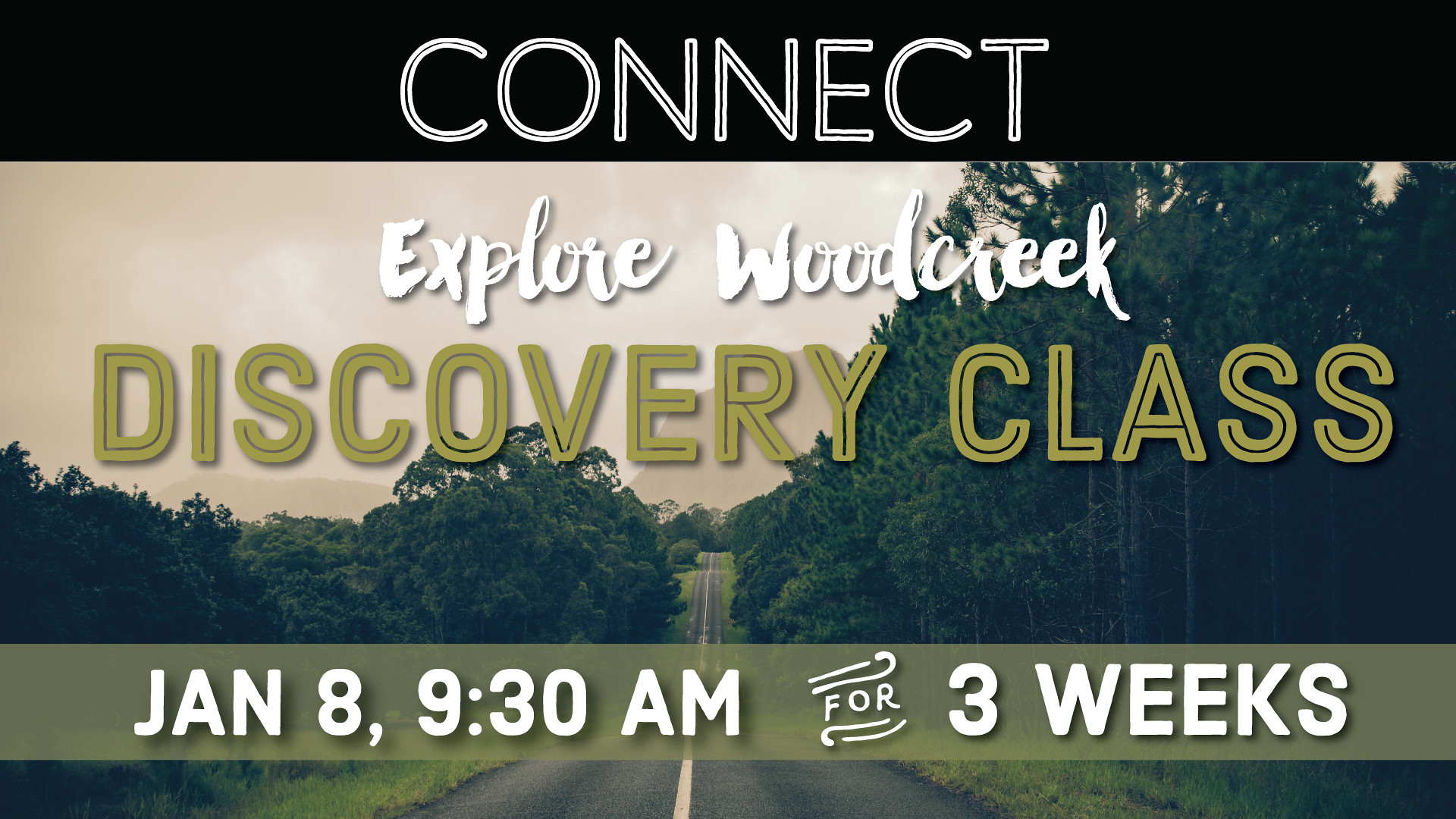In this black-and-white, landscape-oriented image, the central subject is a single-lane road stretching from the bottom center towards the horizon, flanked by lush green grass and trees with bushy leaves. The trees and grass create a natural border on either side of the road. Hills are visible in the background, and the sky above has a light brown or foggy appearance, featuring some clouds.

The image features informative text about an upcoming event. At the top, a black horizontal band with white text reads "Connect." Below this, superimposed on the photograph, the words "Explore Wood Creek" are written in bold script, followed by "Discovery Class" in all caps and olive green color. At the bottom, another horizontal band—darker green with white lettering—states, "January 8th, 9:30 a.m. for 3 weeks," with decorative flourishes around the word "for."

The photograph combined with graphic design elements gives it an informational and promotional style, suggesting an organized and educational event.